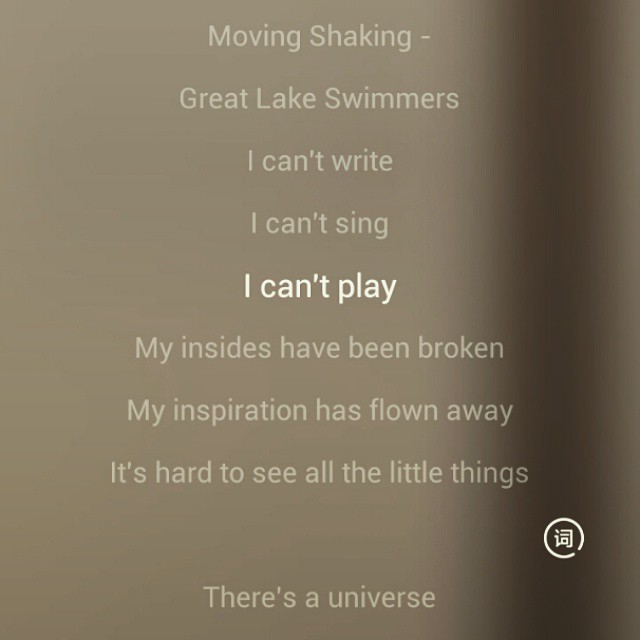This is a cropped photograph of a gray-toned poster displaying a poignant message in varying shades of grey and white text. The poster features the text "moving, shaking, great lake swimmers," followed by "I can't write, I can't sing, I can't play." Further down, it continues with "my insides have been broken, my inspiration has flown away, it's hard to see all the little things, there's a universe." The right-hand side of the poster transitions to a darker grey, nearly black background, bearing a small, unidentified logo resembling an Asian character. This image lacks any identifying information such as date, location, or people, and the text is the central focus.